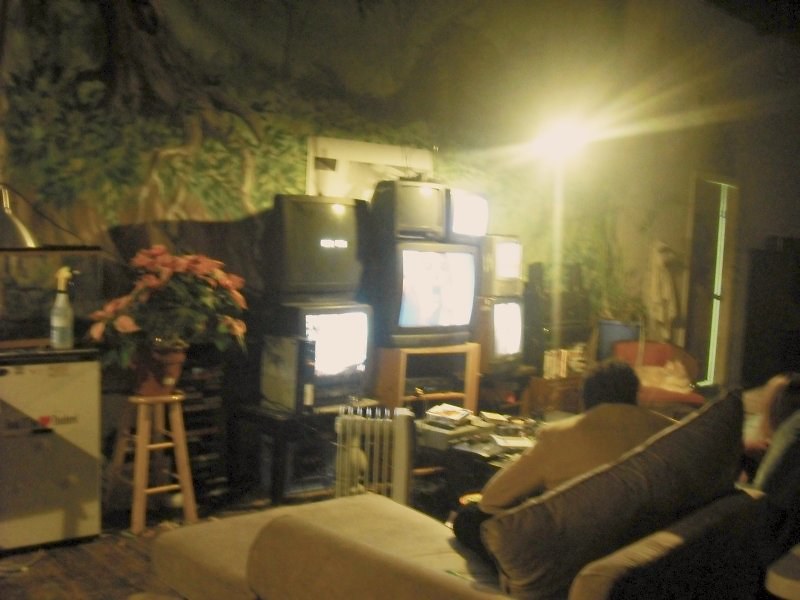The image depicts a dimly lit, slightly blurry room that appears to be a basement or a man cave from decades past. The room is dominated by a wall adorned with a forest-themed mural featuring large trees and green grass. Along this mural-splashed wall, seven CRT TVs of various sizes are arranged on different shelves and tables, with six of them turned on displaying white backgrounds, while one remains off.

In the lower right-hand corner, a man in a long-sleeved white shirt is sitting on an L-shaped white couch, his back facing the viewer. Beside him, the blurred silhouette of another person, possibly a woman with brown hair and a red shirt, is faintly visible. To the left of the TV arrangement stands a wooden stool holding a large orange pot filled with green leaves and pink flowers. Adjacent to this is a small fridge, on top of which rests a nearly half-full bottle with a nozzle cap and a water bottle.

The upper right quadrant of the image is marred by a bright, star-burst-like glare from a light, which spreads its beams across the scene, contributing to the image's overall lack of focus. Other elements in the room include a white radiator heater, a mattress on the floor, and a table cluttered with various papers. A slightly ajar door can be seen in the background, further adding to the room's cluttered and somewhat nostalgic ambiance.